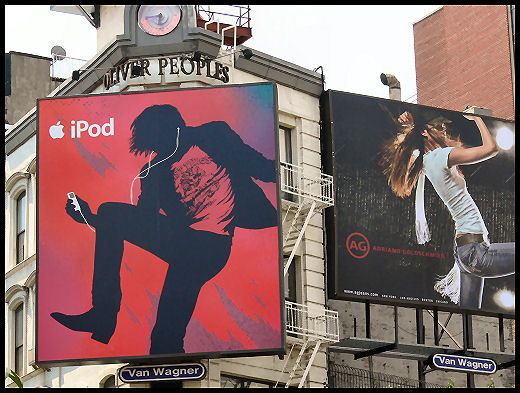The photograph features a bustling urban scene dominated by advertisements. Centered prominently is a white building, possibly an apartment complex, with "Oliver Peoples" written in modest lettering at its top. Affixed to the center of this building is a massive rectangular billboard obscuring a significant portion of the facade. The billboard is vivid red, showcasing the iconic white iPod held by a black silhouette character, with white earphones clearly leading up to the figure's ears, amplifying the ad's impact. To the right of this building stands another billboard. This one features a person with long hair, dressed in a white top and gray pants, outlined in black. Although the text on this sign is not readable, the careful layering and bold outlines make the figure stand out against the urban landscape. Together, these layered advertisements create a striking visual interplay, embedding commercial culture deeply into the city’s architectural fabric.